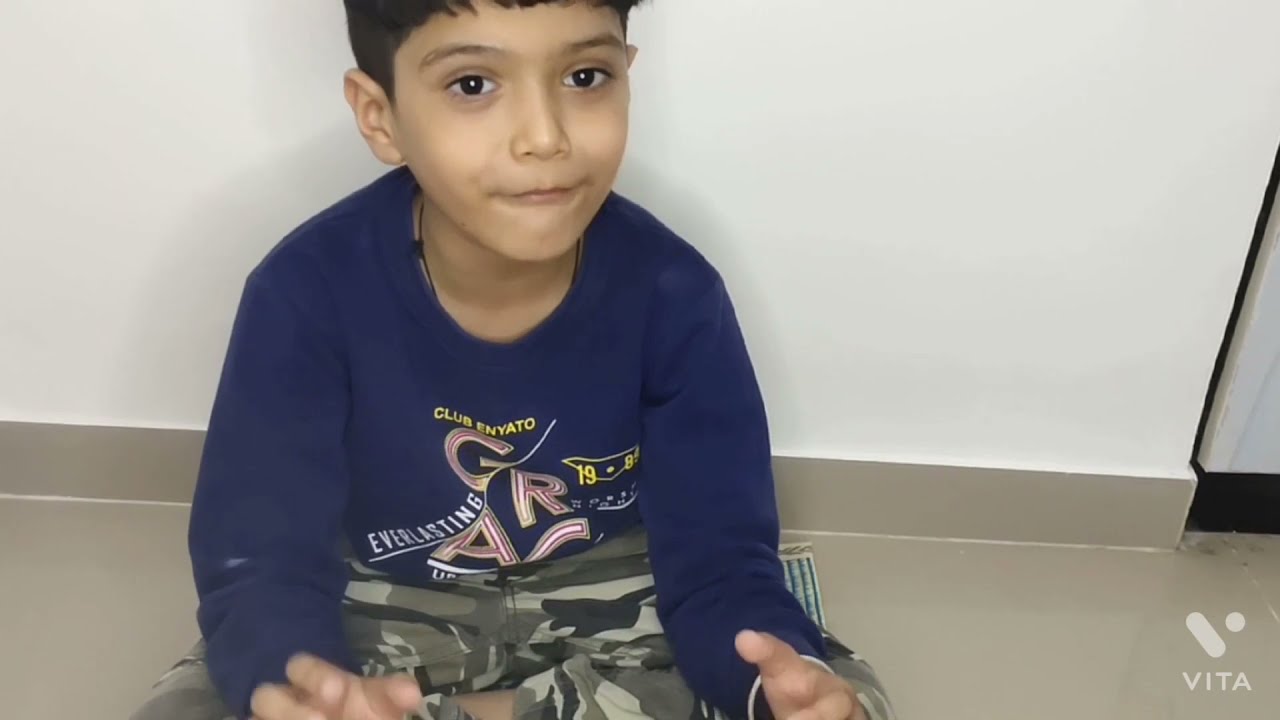The image captures a young boy, likely between five and seven years old, seated cross-legged on a beige floor, possibly made of cement. He is positioned against a white or cream wall with a grayish-tan molding at the bottom edge. The boy has short, dark brown hair and dark brown eyes, and his skin is a brown tone. He is looking slightly past the camera with a subtle smirk or pursed lips, as if sucking on hard candy. The boy is dressed in a long-sleeve dark blue sweatshirt that features the words "Club Enyato" in yellow and "Everlasting" in white, among other partially obscured graphics. He pairs this with green camouflage pants. A mat is partially visible at the bottom right of the image, along with a small icon that reads "Vida."